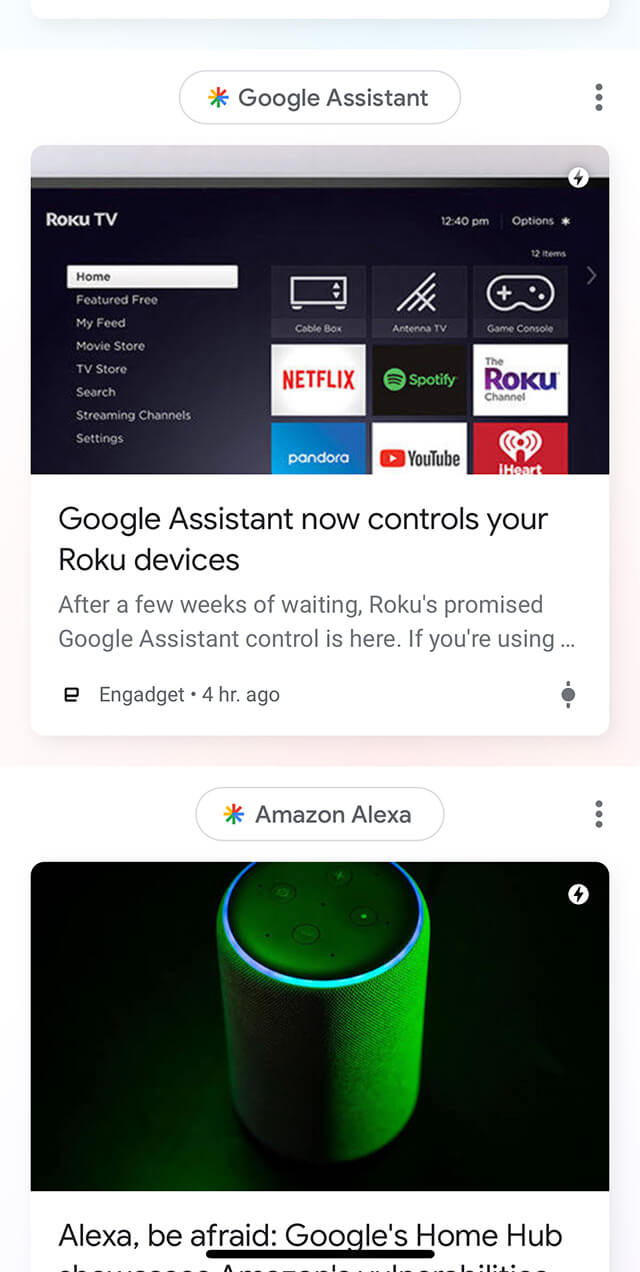The image is a composite screenshot from a website, structured into two distinct panels.

The upper panel features a clean, white background with centered text reading "Google Assistant" in bold letters, accompanied by the initials 'GA'. On the right side of this text are three vertically aligned dots, suggesting additional options. A transparent gray banner runs across the top of this panel, lacking any discernible content.

The lower panel contrasts with a black background. In the upper left corner, the text "Roku TV" and the time "12:40 PM" are displayed, with the word "Options" nearby. Below, a vertical menu lists various categories: "Home," "Featured Free," "My Feed," "Movie Store," "TV Store," "Search," "Streaming Channels," and "Settings." Adjacent to this menu, twelve item icons represent popular streaming and multimedia services, including Netflix, Pandora, YouTube, Spotify, Roku, iHeart, Game Console, Antenna TV, and Cablebox. A caption beneath these icons announces, "Google Assistant now controls your Roku devices."

At the bottom of this panel, the image of an Amazon Alexa Home Hub is partially visible with text that begins "Alexa, be afraid..." but is cut off, hinting at a comparison or contrast between the Google and Amazon smart home devices.